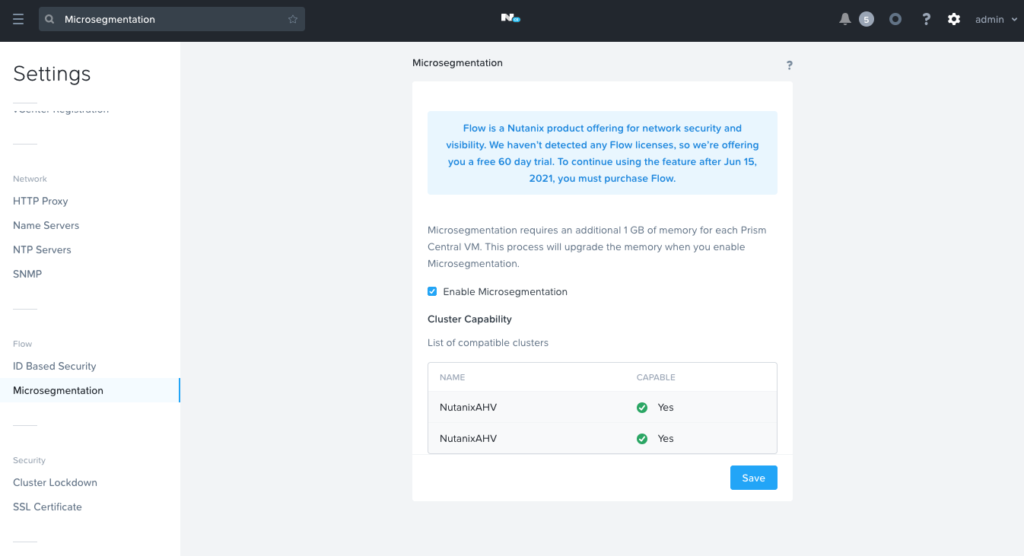A screenshot of a business software interface shows a sleek, modern design with a black navigation bar at the top. The navigation bar features a minimalistic logo: a white letter **"N"** followed by a dot. Just to the left of this, a search bar displays the term **"micro-segmentation"** that has been entered by the user. 

Below the search header, the main section elaborates on the search term, explaining the product offering: **"Flow"** by Nutanix. The description highlights Flow as a product designed for network security and visibility. A notice below the description mentions that no Flow licenses have been detected on the account, prompting an offer for a free 60-day trial. To activate the trial, users need to check a nearby checkbox labeled **"Enable micro-segmentation"** and then click the **"Save"** button to finalize the setup.

The left sidebar features a clearly organized navigation menu, divided into distinct sections titled **"Network,"** **"Flow,"** and **"Security."** This structured layout assists users in navigating through various features of the business software, with a primary focus on enhancing network security through micro-segmentation. The interface reflects a user-friendly approach, facilitating efficient activation and management of security features.